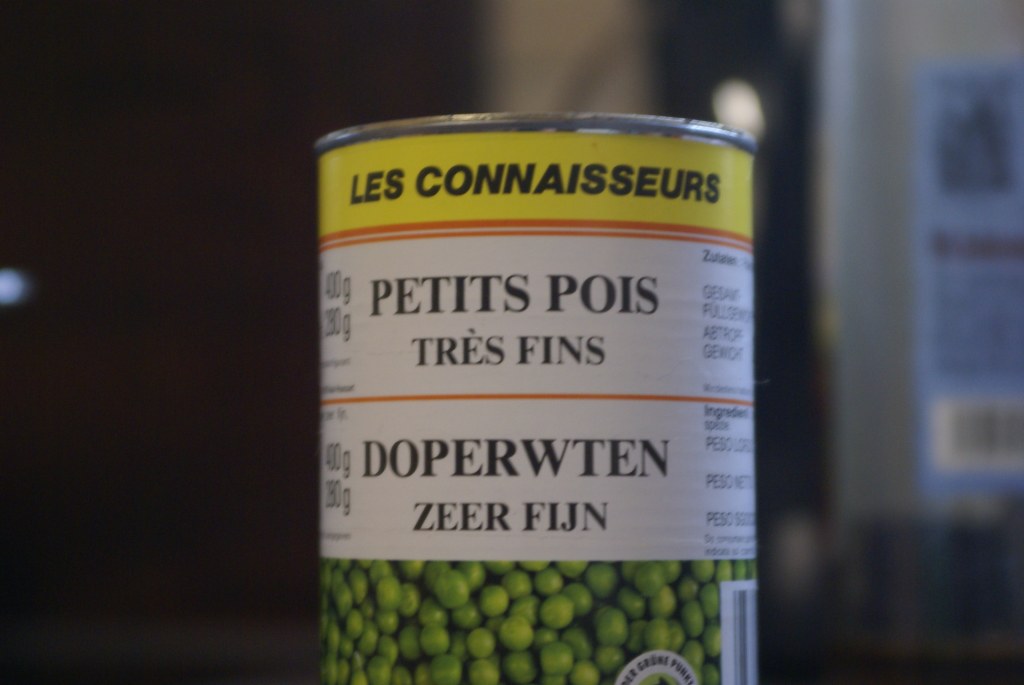This photograph showcases a can of peas, centrally placed against a stark background. The left side of the background is completely black, while the right side is so blurry that it becomes indecipherable, though one can make out a light blue logo with a barcode, suggesting some form of packaging. The can itself is a standard type used for packaging vegetables or similar items.

The can's label prominently features text in at least two different languages. At the top, a yellow stripe with bold, all-caps black font reads "Les Connoisseurs." At the bottom of the label, a photograph of peas is displayed, clearly indicating the can's contents. Below this image, there are two white stripes containing text in different languages. The upper white stripe text reads "Petit Pois Très Fin," which is French. The lower stripe likely contains text in another language, possibly Swedish, though it is not attempted to be pronounced in the description.